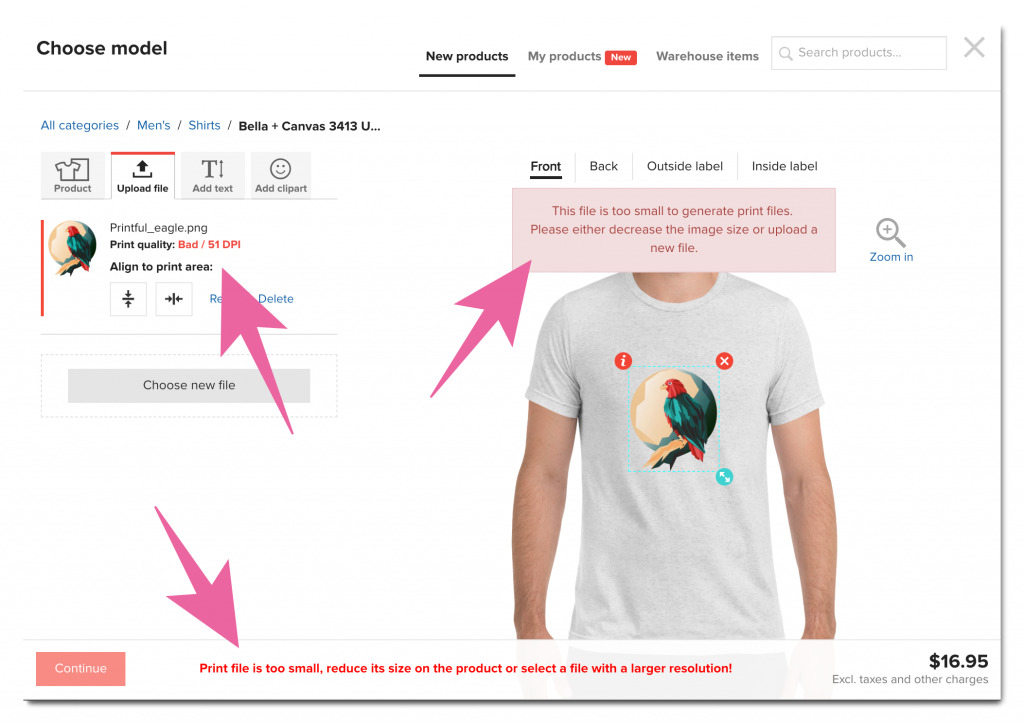This detailed caption is for an image that depicts a screenshot of a webpage used for customizing products:

At the top left corner of the webpage, the text "Choose Model" is displayed. Next to it, the menu includes options labeled "New Products," "My Products," and "Warehouse Items." The "New Products" option is highlighted and underlined, accompanied by a small red "NEW" box. In the upper right-hand corner, there's a "Search Products" box with an adjacent "X" button.

Below the menu bar, the navigation path reads "All Categories / Men's / Shirt / Bella + Canvas 3413U..." Beneath this, there's an image of a man's torso wearing a T-shirt featuring a vivid graphic of an exotic bird, likely a parrot, perched on a branch with a sunset in the background. Surrounding the graphic is a turquoise box, suggesting options to adjust and reposition the image. At the top left of the image, an icon with an information circle is visible, while an "X" circle can be seen on the right. The bottom right of the turquoise box contains an icon with two arrows, indicating the option to expand the image.

A notification at the bottom of the screen states: "Print file is too small. Reduce its size on the product or select a file with larger resolution." On the right side, the price "$16.95" is displayed. The left side of the screen features a panel with options to "Make Your Product," "Upload a File," "Add Text," and "Add Clip Art." Pink arrows are strategically placed to indicate that the current image size is incorrect for the upload.